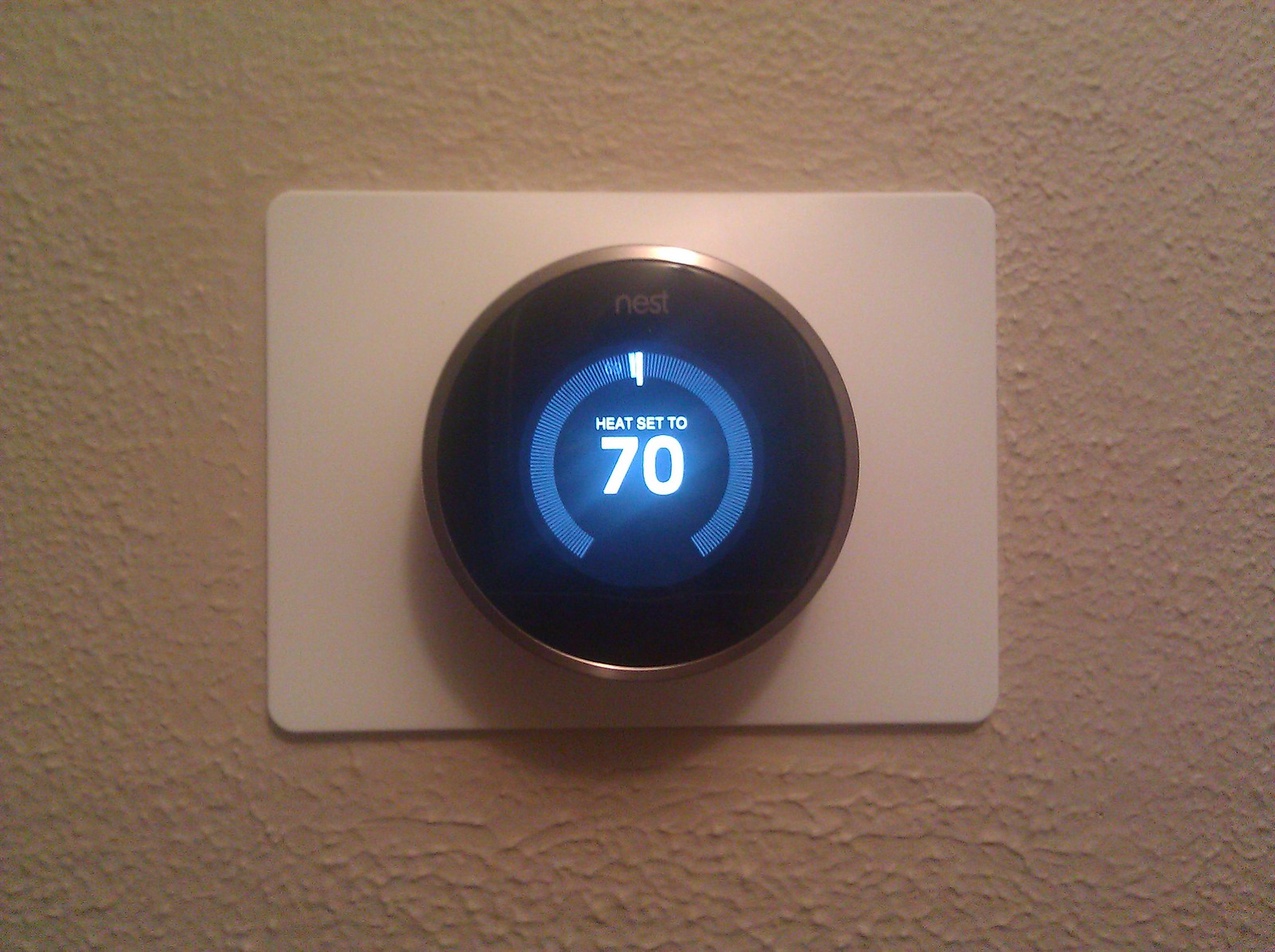This image features a modern Nest thermostat mounted on a wall. The thermostat is installed on a square, white plastic base that is affixed to a textured, white-painted drywall surface, indicating it's an older wall with a thick texture. The Nest thermostat itself is round, with a sleek silver exterior border. The inner display is black with the brand name "Nest" prominently displayed at the top in gray lettering. The central part of the thermostat is illuminated with a blue background, and light blue slashes form a halo-like pattern. An arrow in white occupies the upper center of the display, pointing towards a specific temperature setting. The display also shows the text "Heat set to 70," glowing clearly in the blue-lit background.